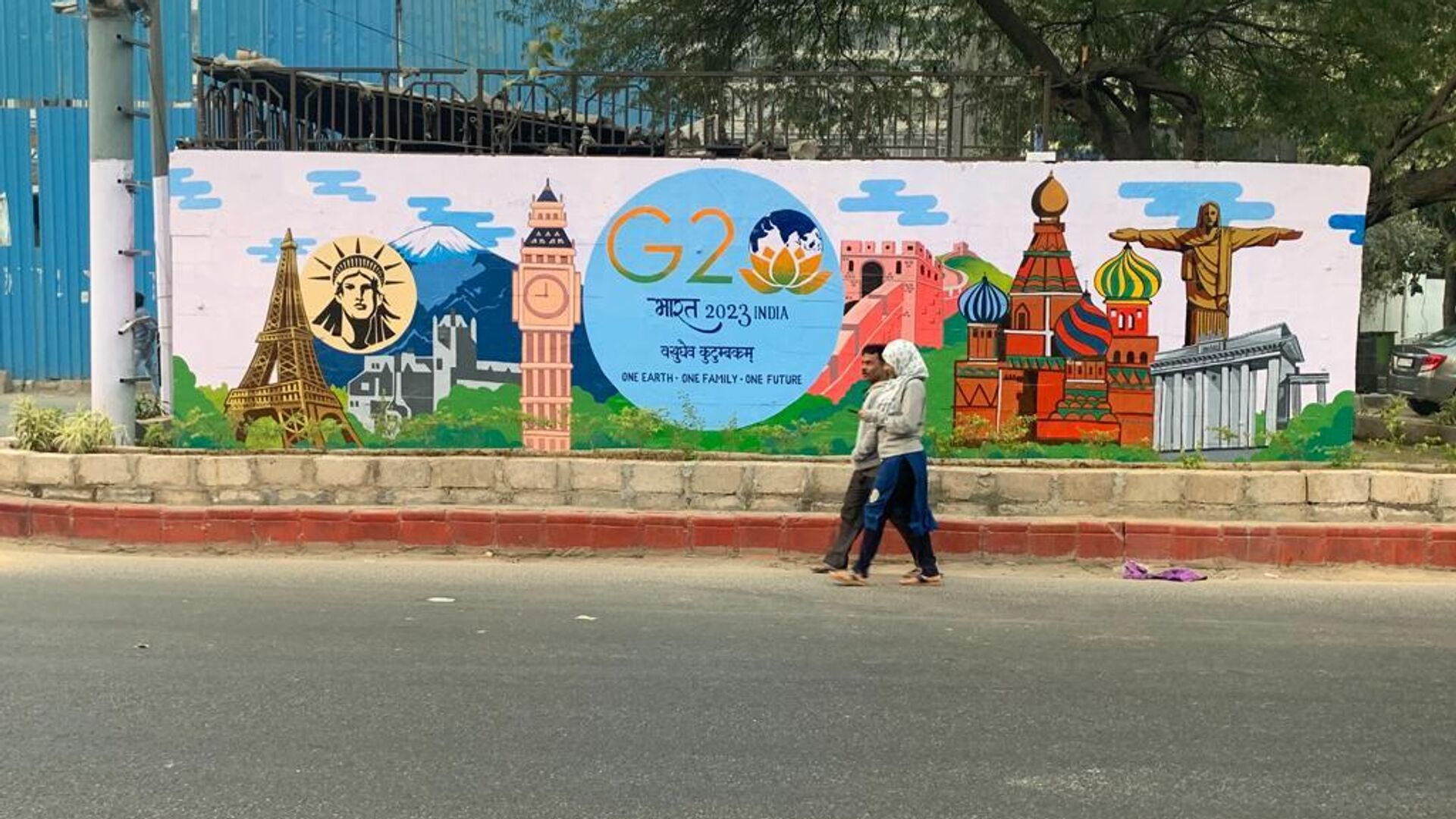This daytime street scene photograph captures a vibrant mural on a large concrete wall. In the center of the frame are two individuals walking from right to left: a man in a gray hoodie and dark pants with brown hair, and a woman closer to the camera wearing a white head wrap, gray long-sleeved shirt, black pants, and brown sandals. The man walks on the far side of the street, while the woman, who also has a blue coat tied around her waist, is closer to the camera. The street they walk on is dark black, creating a stark contrast to the vivid mural behind them.

The mural, which stretches across nearly the entire picture, features various iconic landmarks and cultural symbols from around the world. On the left, the Eiffel Tower gleams in gold, and nearby, a coin with the Statue of Liberty's face is prominently displayed. Below and to the left, there's a gray castle with Mount Everest towering in the distance, its blue and white peak clearly visible. Big Ben is depicted next to these landmarks. 

At the center of the mural, a large blue circle contains the text "G2 2023 India" in bold yellow and green letters, signifying a global theme. To the right of the circle, the Great Wall of China ascends a green mountain, followed by the Taj Mahal facing the viewer. Further right, the Roman Coliseum stands tall with a golden statue of Jesus with outstretched arms behind it. Green grass lines the bottom of the mural, adding a touch of natural beauty to the scene. 

The photo also includes environmental details: thin stacks of orange bricks and a concrete barrier in the foreground, blue metal containers lining the background, and a big green tree along the right side. A power pole, white halfway up shifting to gray, stands prominently on the left, adding to the urban landscape's authenticity.